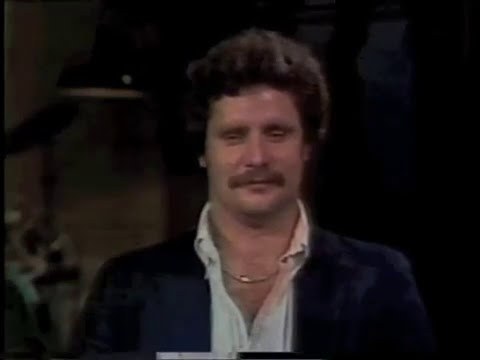The image appears to be a still from a TV show or video, likely from the 70s or 80s, featuring a Caucasian man around 40 years old. He stands at the center of the slightly wide, rectangular frame, the dark background primarily black with hints of brown light and a wood-paneled wall on the left. The man has a small brown afro and a caterpillar-style mustache, and he's gazing downward with a slight smile, his eyes barely open. Dressed in a shiny navy blue, possibly black, dress jacket over a white collared shirt unbuttoned at the top, he also sports a gold necklace. His shoulders and upper torso, along with the lower part of his ears, are visible, and his head occupies the top half of the image. The scene has a studio-like ambiance, reinforcing the impression of a snapshot from a television episode.